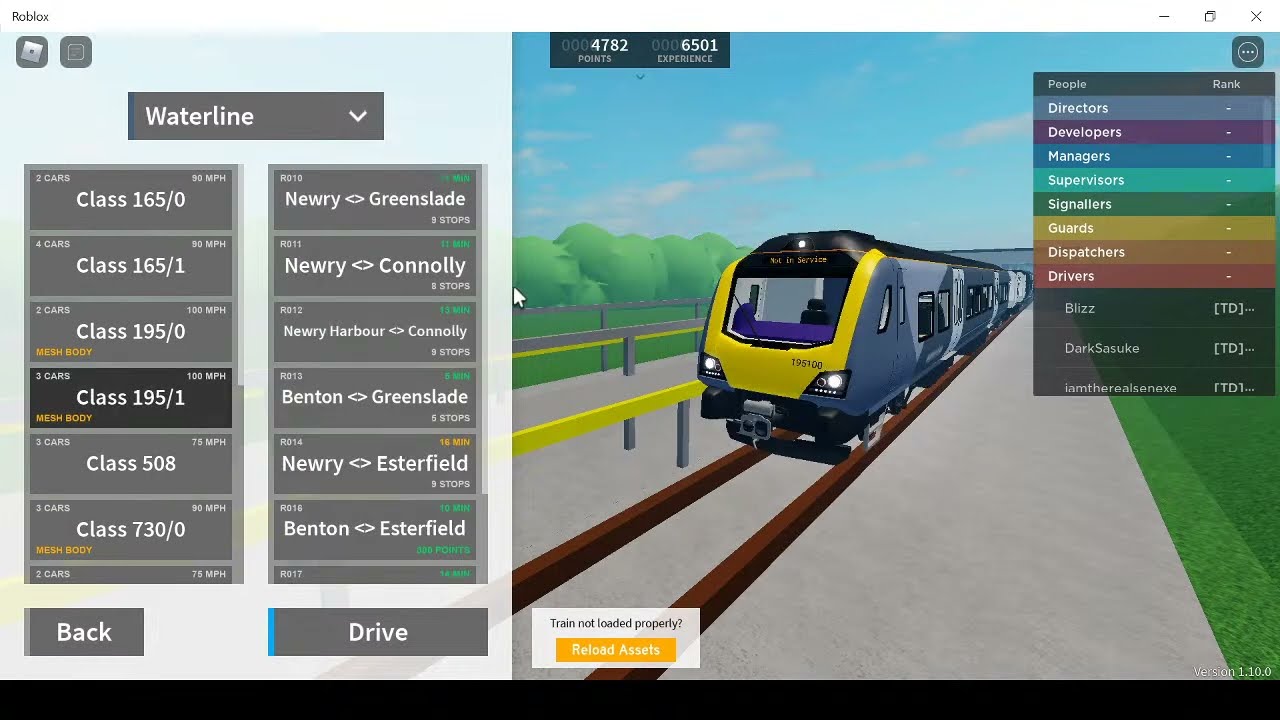The image is a screenshot of a computer application that appears to be a train or rail system interface, possibly for schedules or train management. The application is divided into two main sections. On the right side, there is a low-polygon, 3D rendering of a train, placed on a red track situated on a gray concrete floor. Surrounding the scene are lush green grass on the right and tall trees on the left, under a partly cloudy blue sky. The train itself features a yellow front with operational headlights, a black roof, and a distinctive urban camo pattern of mixed gray and blue shades. The front includes a large window, and there are smaller windows along the sides. Inside, the cabin has a blue dashboard and a black chair.

On the left side of the application, there is a text chart. At the top of this section, a drop-down box labeled "Waterline" is visible. Below this are two columns. The left column lists various train classes and their specifications, such as "two cars, class 165-0, 90 miles per hour," "two cars, class 190-0, 103 miles per hour," and others including class 195-1, class 508, and class 730. The right column lists destinations and routes, such as "Newry to Greenslade," "Newry to Connolly," "Newry Harbor to Connolly," and "Benton to Greenslade." Each entry in this column is highlighted in a different color of the rainbow, adding a vibrant visual element to the information displayed.